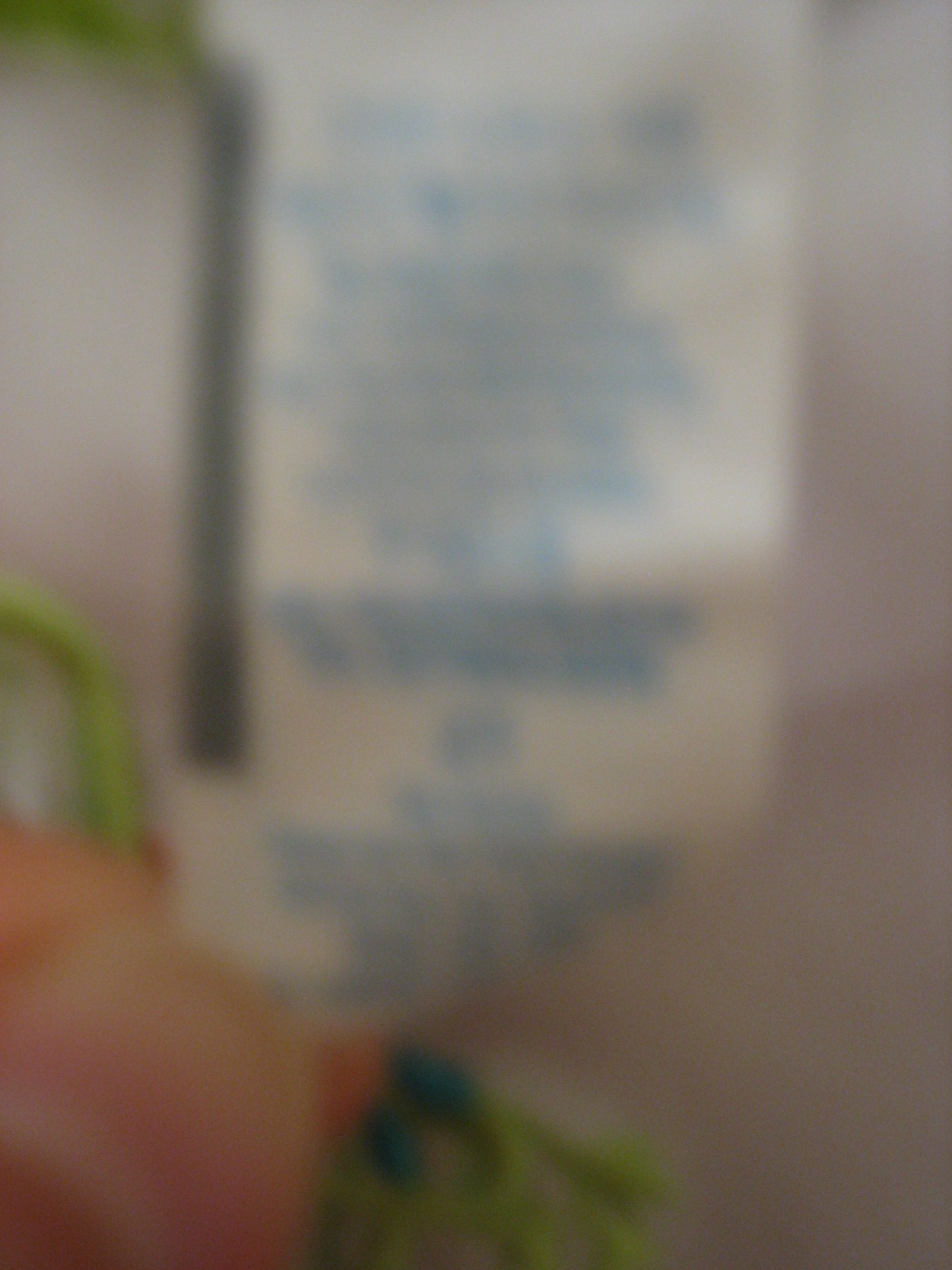The image is a blurry photograph featuring a predominantly white background that becomes progressively shaded and darker toward the bottom. In the bottom left corner, there's an indistinct orange object with two green items extending from it—one on each side. The top left quadrant of the image contains another green element. Centrally located is a white, rectangular shape marked by a black vertical line along its left edge. This rectangle features blue text stretching from the top to the bottom edge, seemingly organized into multiple lines or potentially several paragraphs, extending down towards the orange object at the bottom.